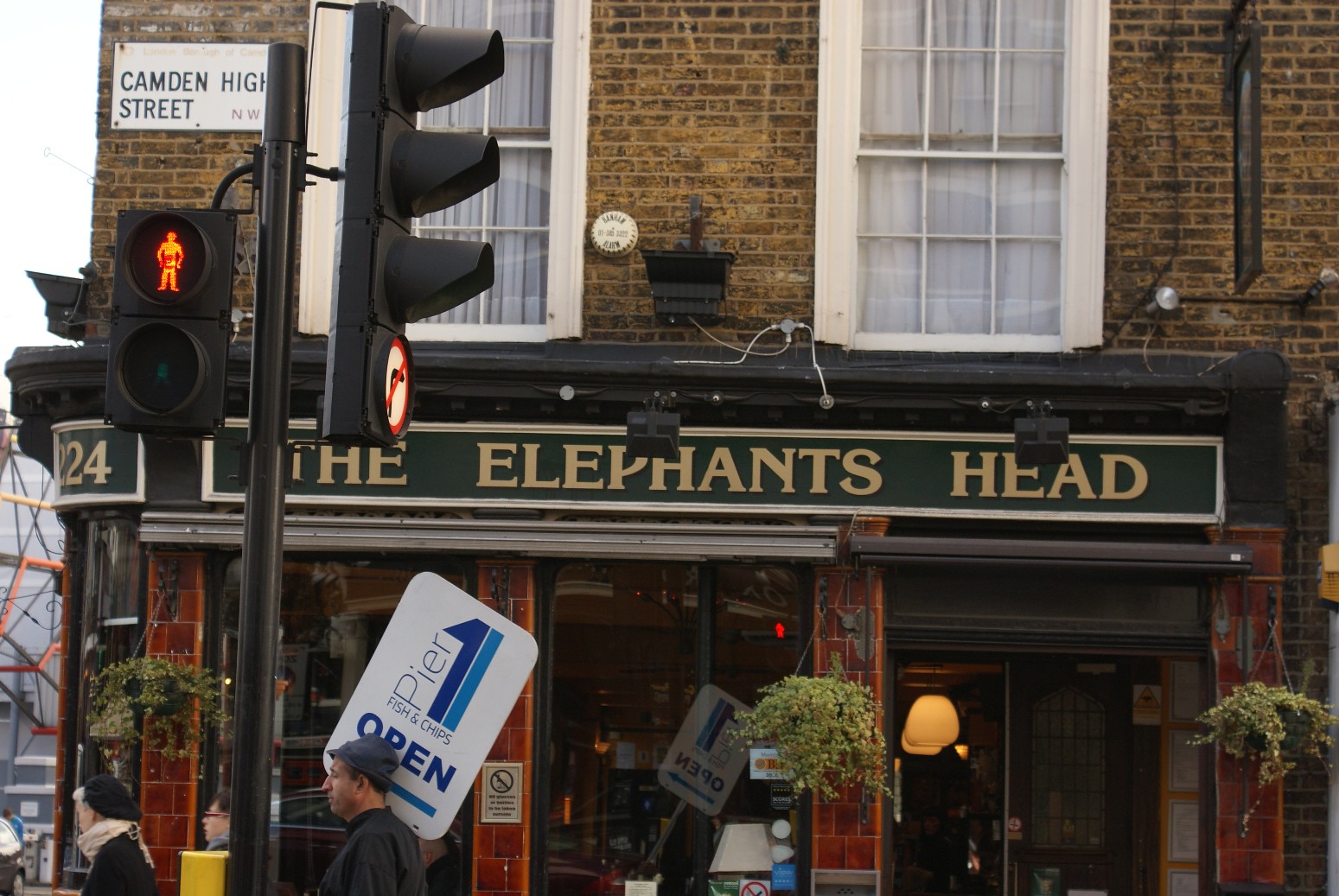This photograph captures the bustling atmosphere of a street corner on Camden High Street, featuring the prominent storefront of The Elephant's Head, a pub housed in a distinct brown brick building with scratchy beige marks. The top of the ground floor is adorned with a bold, black sign with tan capital letters spelling out "THE ELEPHANT'S HEAD." White-framed windows punctuate the facade, adding a touch of contrast to the rustic exterior. Below the sign, the entrance is visible, hinting at the establishment's inviting interior.

In the foreground, two pedestrians animate the scene. A man in a black hat and black t-shirt strides by, holding a large white sign that reads "PIER 1 OPEN." Nearby, a woman, also in a black hat adorned with a white scarf and matching black top, walks purposefully. Additional details include a metal pole with a stop sign and a sans-serif black-font sign declaring "Camden High Street NW" in the top left corner of the image, further anchoring the photo in its vibrant urban setting.